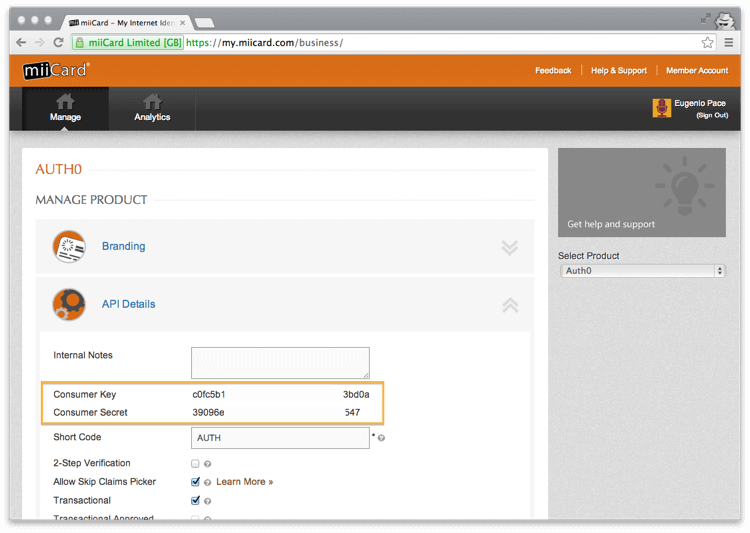This is a detailed screenshot of a browser window that resembles a macOS interface but differs in a few key aspects. At the top left corner, there are three circular buttons typically colored red, yellow, and green in macOS, but in this instance, they are white. The browser window has a gray frame which suggests it might be a different or modified operating system.

The address bar indicates that the site being viewed is "MiiCard Limited GB" with a green padlock icon, suggesting a secure connection. The URL displayed is "https://my.miicard.com/". At the top of the webpage, there's an orange strip featuring the MiiCard logo: the word "me" in small letters on a black rectangle, followed by "Card" with a capital "C".

Towards the upper right of the webpage are options labeled "Feedback," "Help and Support," and "Member Account." Below this is a gray navigation strip with tabs for "Manage" and "Analytics," with the "Manage" tab currently active. 

Within the "Manage" tab, there is a highlighted pop-up window that begins with "AUTHO" where the "O" might be a zero. This pop-up is titled "Manage Product" and includes two sections: "Branding" and "API Details." The "Branding" section is collapsed while the "API Details" section is expanded.

The content of the "API Details" section includes internal notes, currently displayed in a blank text box. There is a highlighted golden yellow rectangle around the area showing "Consumer Key" and "Consumer Secret," followed by sequences of numbers and letters that are difficult to read due to their size. Below this, there is another text box labeled "Short Code" which contains the text "AUTH."

Further down, there are additional settings including "Two-Step Verification" with an unchecked box, "Allow Skip Claims Picker" with a checked box, and "Transactional" also with a checked box.